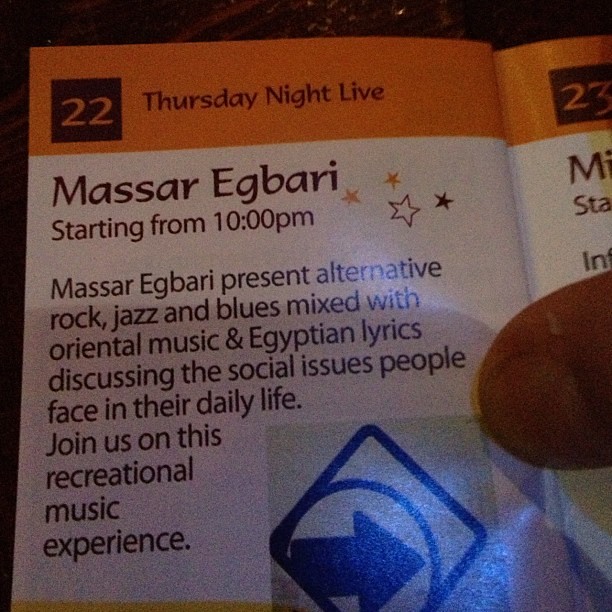The image depicts a pamphlet being held down by a person's finger at the middle right. At the top left, the pamphlet features an orange banner with black text reading "Thursday Night Live." Positioned next to this is a black square with orange text displaying the number "22." Below this banner is white space containing detailed event information: "Massar Egbari, starting from 10 p.m. Massar Egbari present alternative rock, jazz, and blues mixed with Oriental music and Egyptian lyrics discussing the social issues people face in their daily life. Join us on this recreational music experience." The bottom right corner of this page showcases an arrow pointing right, encased in a circle within a diamond shape. This design element is situated inside a green square. Additionally, there are four stars on the right side: one white, one orange, a lighter orange, and one black. Slightly visible on the opposite page is the number "23" and partial letters "MI," suggesting continuation or another event.